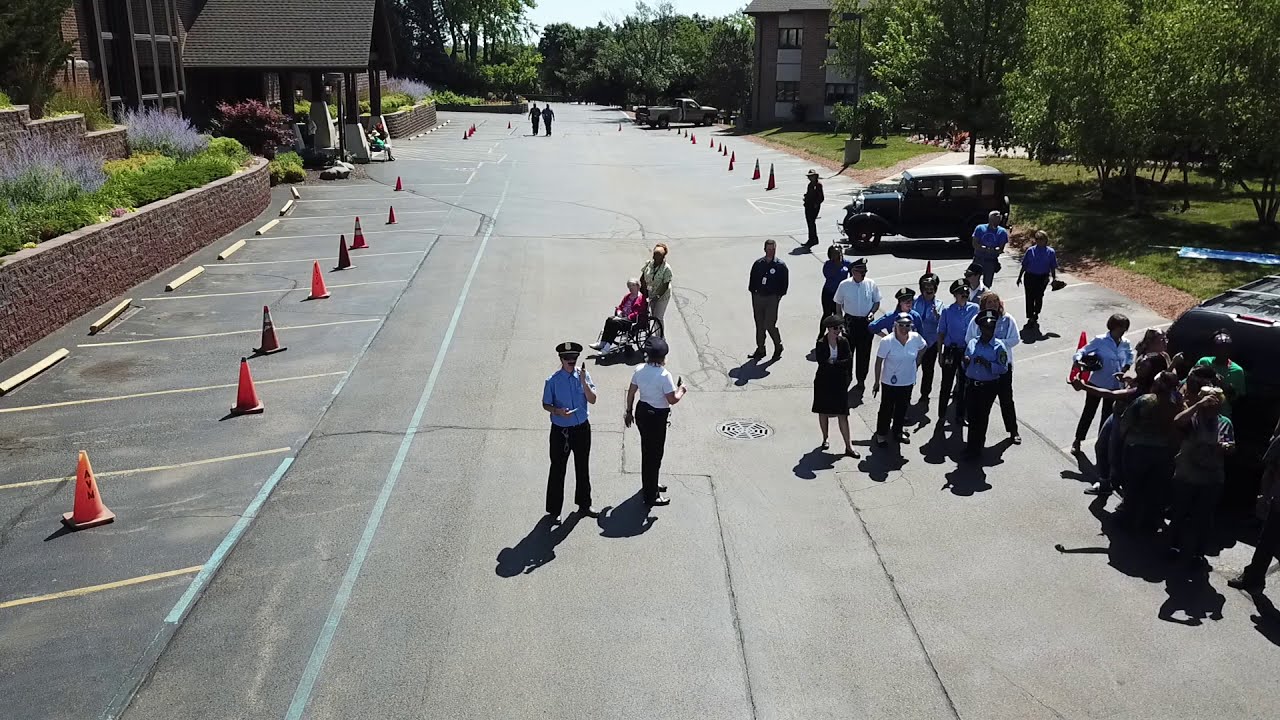This aerial color photograph captures a street scene on a bright, sunny day, possibly on a college campus. The image is taken from above, revealing a well-paved road running down the center, flanked by green trees and grassy areas. The foreground is dominated by approximately two dozen people, many in police uniforms with blue shirts, caps, and dark pants. A notable figure in a police uniform stands prominently near the center, holding something in his hands. Orange traffic cones block the white-lined parking spaces to the left, signaling restricted access. On the left side of the street, a brown brick building curves into view, while two more dark brown buildings are visible on the right amidst large green trees. A person is seen pushing a wheelchair, adding to the scene's dynamism. Towards the background, an old-style jeep and a truck are parked on the right, and the road eventually disappears into a verdant horizon lined with more trees. The photograph, distinguished by its realistic and representational style, offers a comprehensive and detailed portrayal of the bustling outdoor scene.